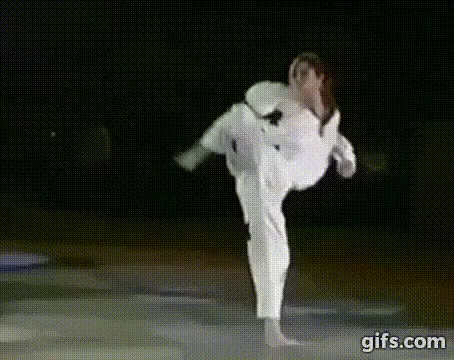This is a photograph of a white woman with long brown hair performing a high karate kick. She is wearing a traditional white karate outfit and appears to be barefoot, standing on a gray floor against a solid black background. The image, though blurry, carries the watermark "GIFS.com" in white letters with a black border at the lower right-hand corner, suggesting that it could originally be part of an animated GIF. The woman is planted firmly on her left foot, while her right leg is raised high, almost parallel to the floor. She leans slightly backward with her fists clenched, eyes focused intently on her elevated right foot.